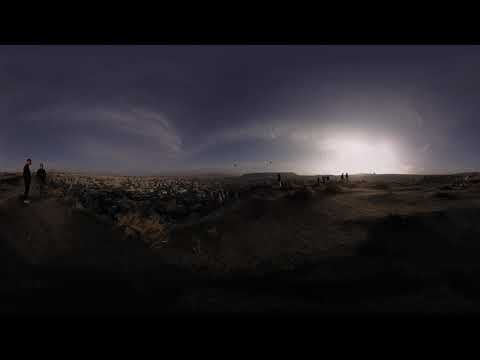The photograph, taken at dusk with a dramatic fish-eye lens effect that distorts the scene into a warped, curvy landscape, presents a captivating view of a desert setting. The sandy ground, with its light tan and brown hues, is dotted with green and yellowish shrubbery. On the left, two men stand on rocks, engaged in conversation, while gazing down at a city below. To the right, more distant figures traverse the top of a mountain, their features indiscernible due to the low resolution and distance. The sky, a darkening blue with wispy white clouds, adds to the twilight atmosphere as the sun sinks just below the horizon. In the muted brown, blue, and black tones of the image, the city—its primarily white, beige, and brown buildings—emerges in the far distance, enhancing the sense of looking out over a vast, serene landscape.